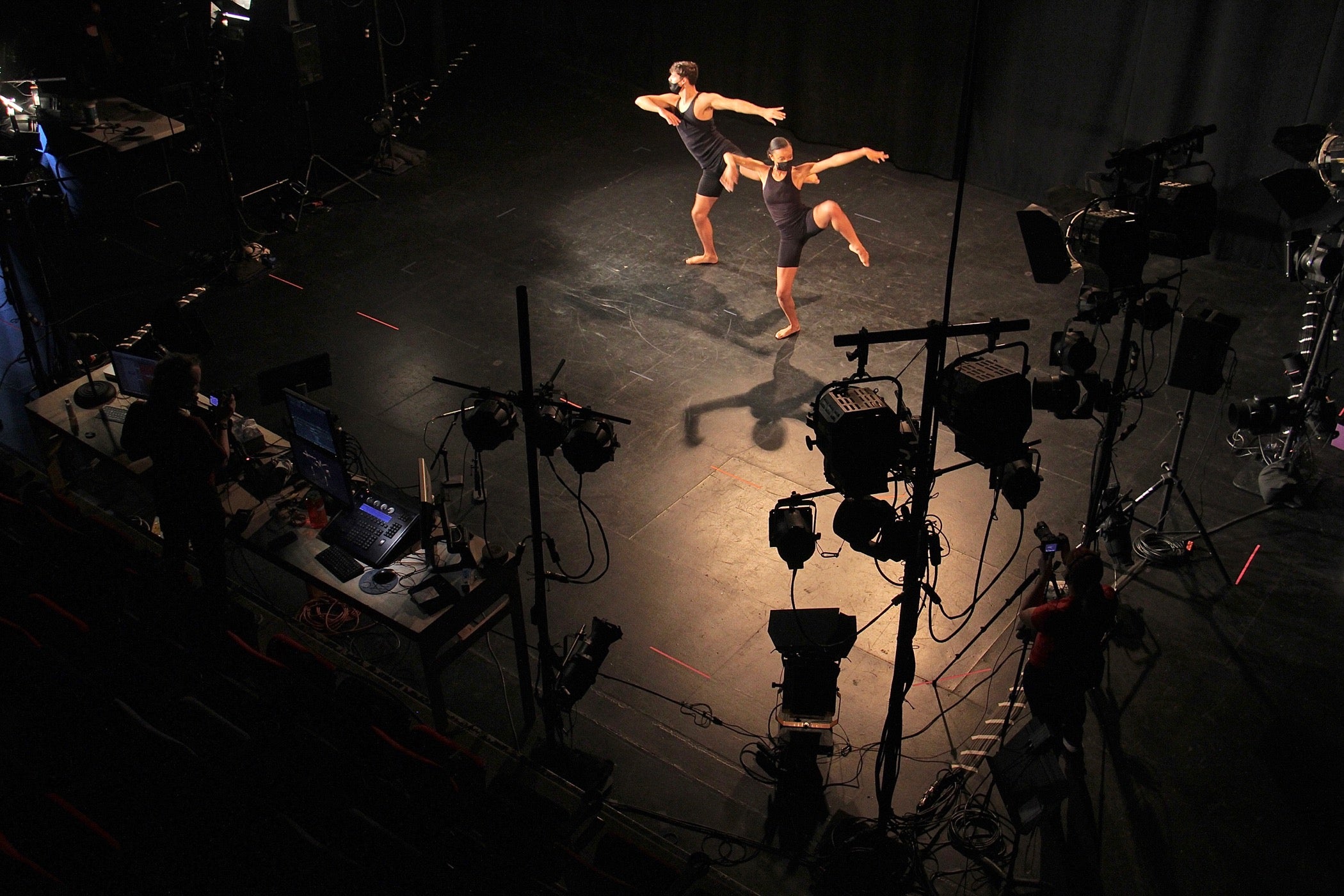In this aerial view of a dimly lit soundstage, two dancers—a man and a woman—are captured mid-performance, striking a crane pose with their left legs raised and arms extended gracefully. Both performers are clad in identical black tank tops, tight black shorts, and black masks, their hair pulled back, with their lighter skin contrasting against their dark ensembles and the black floor. The stage is encircled by cameras and lighting equipment, with a notable figure in a red shirt operating a camera in the bottom right corner. To the bottom left, a production team member stands by a desk cluttered with electronic equipment, computers, and monitors, overseeing the dance. The dancers are illuminated more brightly than their surroundings, emphasizing their central presence amid the otherwise dark and brown-toned stage. Additionally, a few observers can be seen off-stage, engrossed in the performance being filmed.